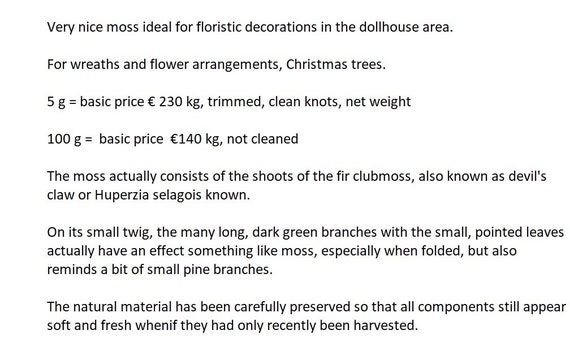Here is a single, detailed caption based on the given inputs:

This image displays black text on a white background, formatted in a clean, sans-serif font. The text reads: "Very nice moss, ideal for floristic decorations in the dollhouse area. For wreaths and flower arrangements, Christmas trees. 5 grams equals the basic price of 230 euros per kilogram, trimmed clean knots, net weight. 100 grams equals the base price of 140 euros per kilogram, knot cleaned." It further explains that the moss actually consists of the shoots of the fir club moss, also known as devil's claw or Huperzia selago. The description highlights that on its small twig, the many long dark green branches with small pointed leaves mimic moss, especially when folded, but also resemble small pine branches. Additionally, the natural material has been carefully preserved to ensure that all components still appear soft and fresh, as if they had only recently been harvested.